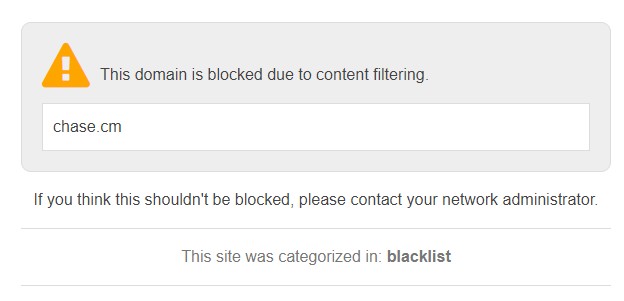The webpage you're attempting to access, chase.cm, has been prevented from loading due to content filtering measures. This domain is currently categorized on a blacklist. If you believe this restriction is in error and that the site should be accessible, please reach out to your network administrator for further assistance and review.